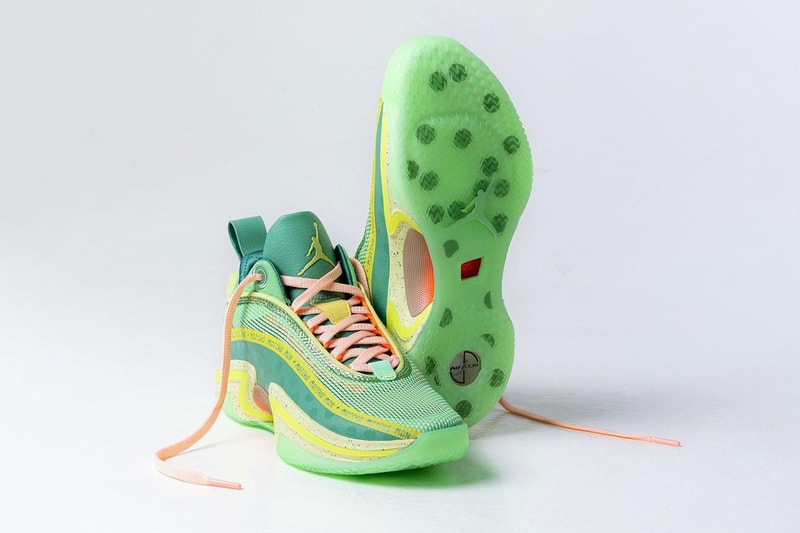The image is a rectangular photograph with a white background, resembling a product photo one might see on a website. It prominently features a pair of Air Jordan sneakers. One shoe lies flat, while the other is propped up to display the sole. The sneakers are a mix of different greens: dark green covers the tongue and back, with light green, almost fluorescent sections, and yellow and white striping along the sides. The soles are a translucent light green with dark green spots and feature a lime green silhouette of Jordan about to dunk a basketball. Both shoes have orange (or peachy pink) laces, which are untied. The tongue displays the Air Jordan logo in white. A red square is situated in the arch area of the soles. The shoes exhibit an intricate design with multiple colors and textures, making them stand out against the stark white background.